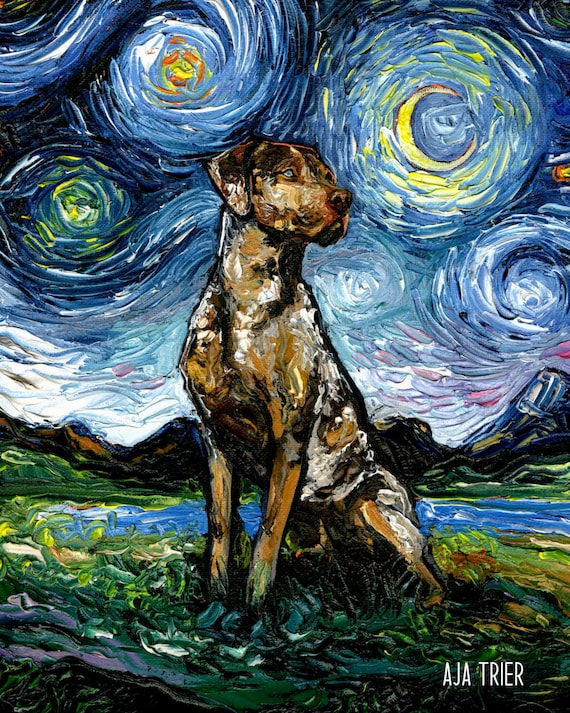This detailed painting by Aja Trier, with her name elegantly printed in a small, artistic sans serif font in the bottom right corner, showcases a brown dog, possibly a Labrador retriever or a setter, sitting regally on a grassy foreground. The dog, distinctively outlined in black and featuring a striking blue eye, gazes to the left. The entire composition is masterfully rendered in the style of Vincent van Gogh's "Starry Night," characterized by swirling, impressionist strokes and a highly textural paint application. The sky is a mesmerizing mix of blues, cool colors, yellows, and a hint of rosy hues, creating the iconic wavy, star-filled backdrop. Behind the dog, a serene body of water lies nestled among dark, shadowy mountains, adding depth to this enchanting outdoor scene. The various shades of green in the grass and the interplay of blue and white in the sky emphasize the painting's dynamic and fluid nature, making it a remarkable tribute to Van Gogh's timeless aesthetic.